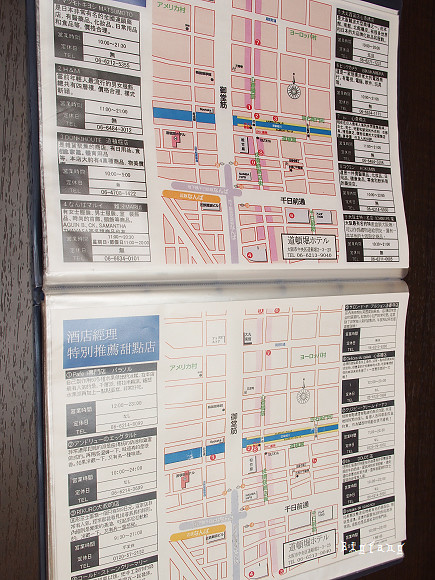The image shows a detailed diagram of a roadway system in an Asian country, prominently featuring a backdrop of dark brown, wood-grain textured walls. The diagram resembles a calendar with two pages, one at the top and one at the bottom, each displaying intricate road structures reminiscent of a Google Maps interface. The top section of the diagram, centered about an inch from the edges, contains a variety of road drawings with paths going in multiple directions, some wider and some thinner, and includes both red and blue blocks indicating different routes. Both sides of this section feature five small squares that provide additional information about the streets. The bottom section mirrors the top with a similar layout of road structures, although the directions of the roads differ. This section, too, has descriptive boxes on both the left and right sides. The diagram appears to be printed in a foreign language, possibly Chinese or Japanese, with pink and white blocks distributed throughout the maps, likely symbolizing different road components or urban areas.